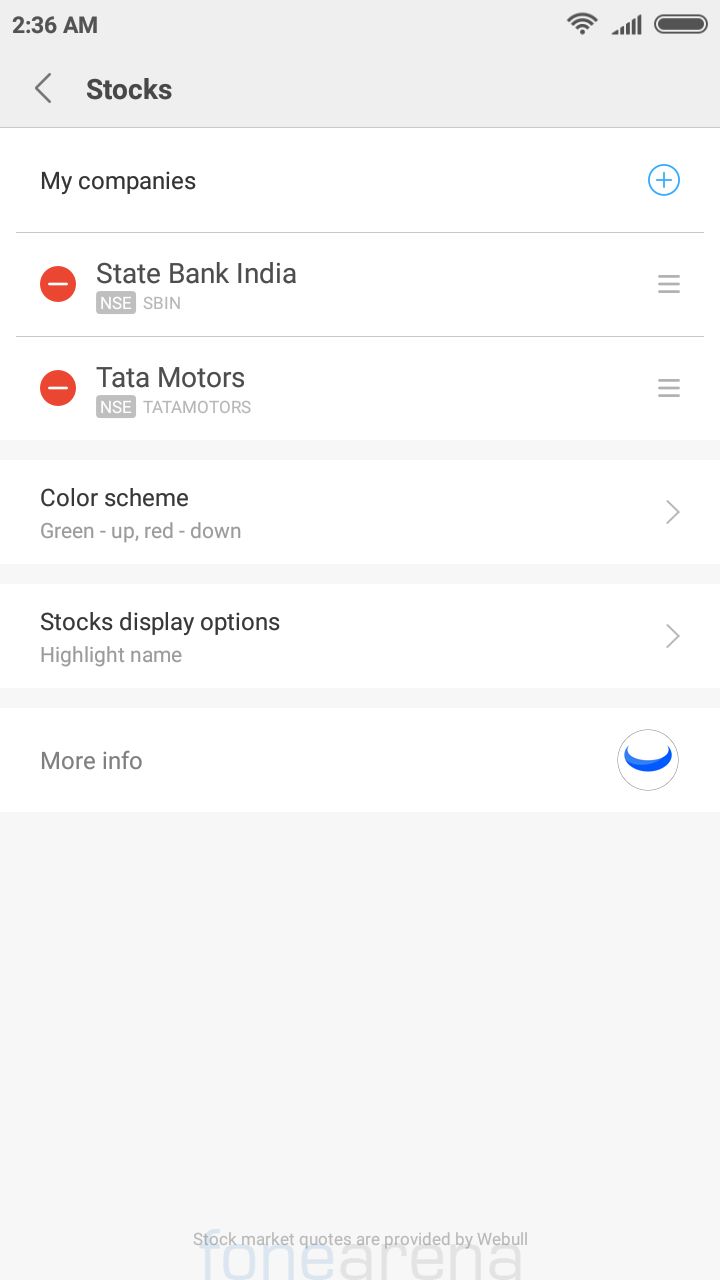The image shows a display entitled "Stocks" on a cell phone or tablet screen. The foremost text indicates that stock market quotes are provided by WEBULL, noted in small print at the bottom of the screen. Behind this information, the larger text reads "TONEARENA." The display lists several companies:

1. **State Bank of India** - Ticker: SBIN, categorized under NSL.
2. **Tata Motors** - Ticker: TATAMOTORS, categorized under NSF.

The display also includes a color scheme where green signifies an increase and red indicates a decrease in stock values. Additionally, an option allows users to highlight the name of the stocks.